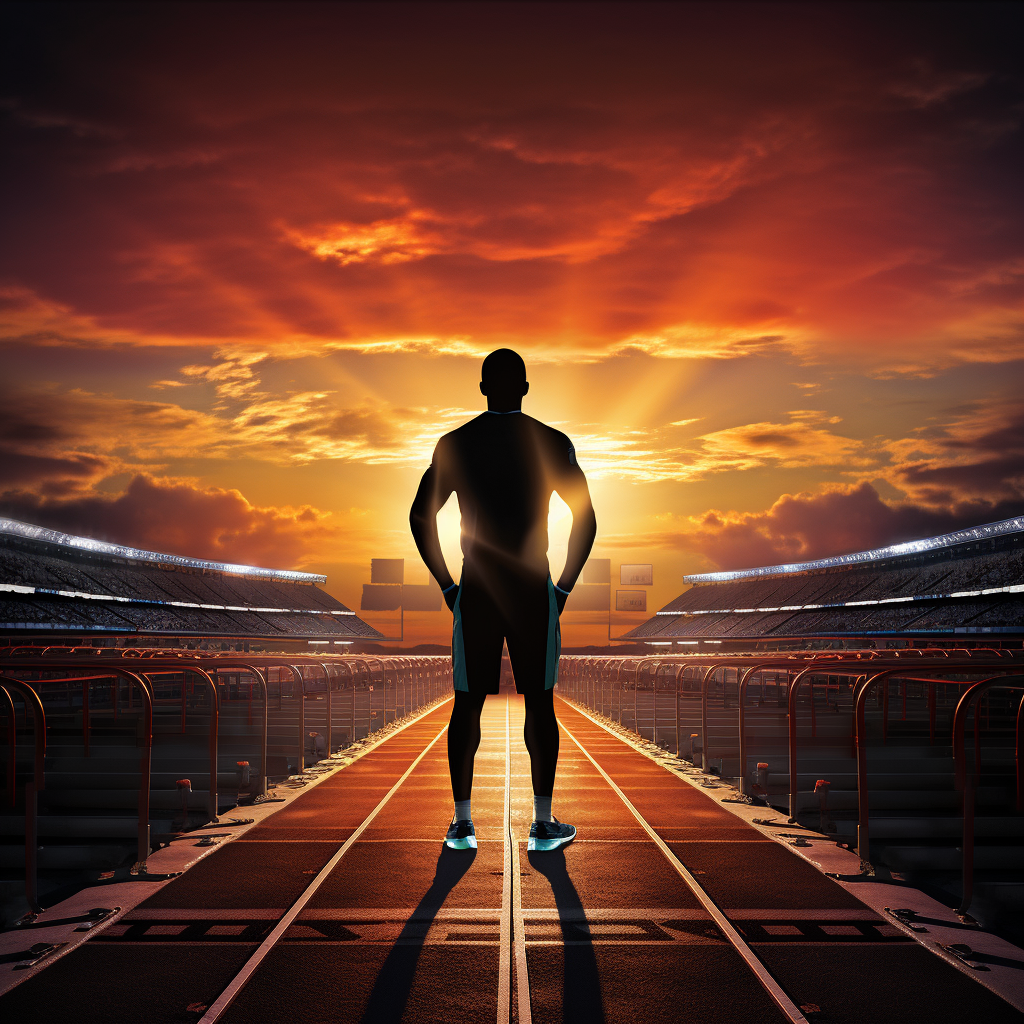In this color animation, an athlete stands on a track lane against a dramatic backdrop of a sunrise. The top of the image features a thick bank of dark orange clouds, with a blue sky and wispy clouds below, illuminated by bright sunlight. The athlete, largely a black silhouette, is centered and facing the sky, resting his hands on his hips. He wears shorts with blue lines on the sides and bright blue shoes. The track lane he stands on is marked by darker brown squares outlined in white, with gate handles on both sides and stands in the far distance. The scene includes AI-rendered details, such as billboards and jump pillars that appear slightly distorted, contributing to a stylized and surreal visual effect.